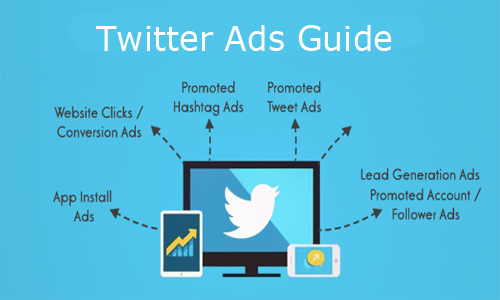The image features a teal-colored background with the title "Twitter Ads Guide" prominently displayed at the top in white print. Situated at the bottom of the image is an animated cartoon illustration of a computer monitor resting on a black pedestal. The monitor screen is black, and in the center, it displays the iconic blue Twitter bird against a white background.

To the left of the monitor, there is a tablet or large cell phone, and to the right, a smaller cell phone is oriented horizontally. The smaller cell phone is adorned with arrows pointing outward from its screen, signifying interaction or direction.

The tablet on the left exhibits stock and bond graphics, while the smaller cell phone on the right features an arrow inside a yellow circle. Encircling these devices are various Twitter ad formats labeled with text:

- Bottom left: "App Install Ads"
- Following clockwise: "Website Clicks/Conversion Ads"
- Top center: "Promoted Hashtag Ads" and "Promoted Tweet Ads"
- Far right: "Lead Generation Ads" and "Promoted Account/Follower Ads"

This composition forms a comprehensive visual guide to the different types of Twitter advertisements available.